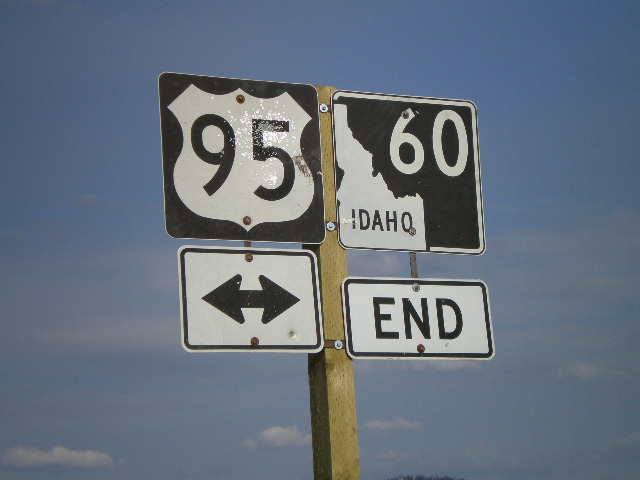This is a high-quality, color photograph of a roadside sign against a clear blue sky with a few white clouds, indicating that it was taken on a beautiful day. The main subject of the photo is a wooden post featuring four metal signs. On the left side, the top sign displays the Highway 95 logo in black and white. Below it, another black and white sign shows arrows pointing left and right, likely indicating directions or exits. On the right side, the top sign features a silhouette of the state with the text "Idaho 60." Below this, a smaller sign reads "End," suggesting the end of the highway or route. The detailed and neatly composed image captures the essence of the roadside signage with the natural backdrop adding to its appeal, making it a potential feature for a travel magazine article about Idaho.